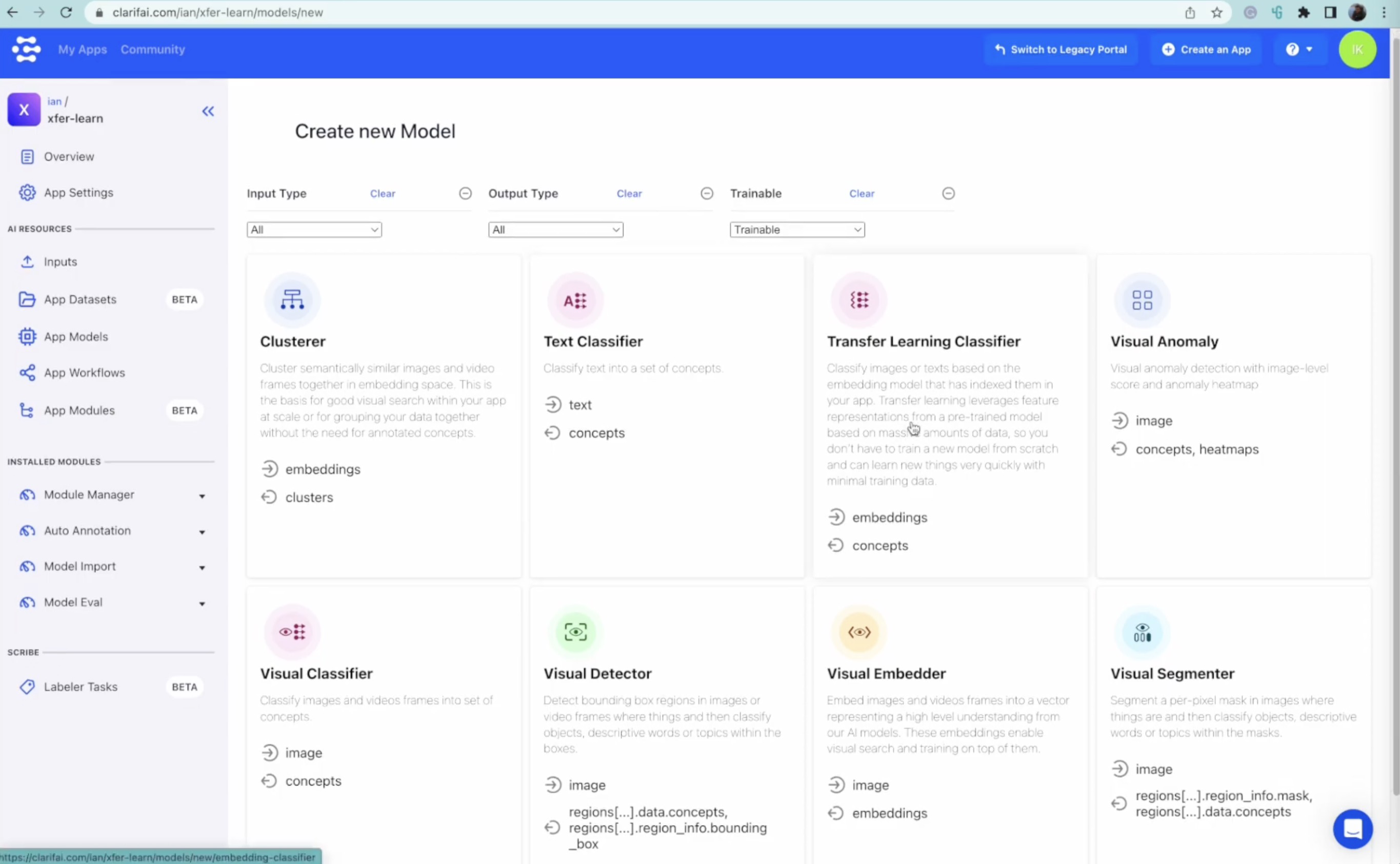**Detailed Descriptive Caption for Web Page Image:**

This image showcases a web page from clarifle.com, categorized under "My Apps Community." The interface features a prominent blue bar across the top. On the left-hand side, a vertical menu lists several options: "Extra Learn," "Overview," and "App Settings." 

Further down, it includes sections for "Inputs," "App Datasets (Beta)," "App Models," "App Workflows," and "App Modules (Beta)." Users can manage various modules and explore features like "Auto Annotation," "Model Import," and "Model Evaluation." 

Additional functionalities include "Labeller Tasks" and creating custom models under the "Create Model" section, categorized by input type, output type, trainability, and specific functions such as "Clusterer," "Text Classifier," "Transfer Learning Classifier," "Visual Anomaly," "Visual Classifier," "Visual Detector," "Visual Embedder," and "Visual Segmenter."

At the top of the page, a green circle likely displaying the initials of the logged-in user is visible. The text throughout the page is notably small and cannot be enlarged.